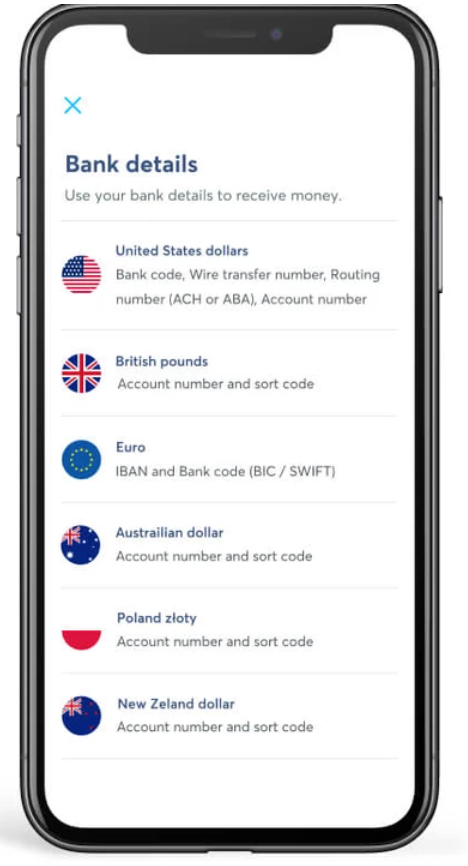Detailed caption: 

The image displays a smartphone against a white background, clearly showing not just the phone screen but the phone itself. On the phone screen, the heading at the upper left is in dark blue text and reads "Bank details," followed by the subheading "Use your bank details to receive money." This appears to be part of a financial application, potentially similar to PayPal, that allows users to receive money in different currencies.

Beneath the headings, there are icons representing various countries paired with their respective currencies and banking information. The breakdown is as follows:

1. United States (American flag icon and "United States Dollars"):
   - Bank code
   - Wire transfer number
   - Routing number (ACH or ABA)
   - Account number

2. United Kingdom (British flag icon and "British Pounds"):
   - Account number
   - Sort code

3. European Union (Euro symbol icon and "Euro"):
   - IBAN
   - Bank code (BIC/SWIFT)

4. Australia (Australian flag icon and "Australian Dollar"):
   - Account number
   - Sort code

5. Poland (Polish flag icon and "Polish Zloty"):
   - Account number
   - Sort code

6. New Zealand (New Zealand flag icon, albeit misspelled as "New Zeland," and "New Zealand Dollar"):
   - Account number
   - Sort code